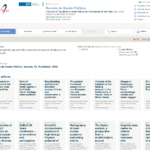A blurry screen capture showcasing what appears to be a webpage with a white background, adorned with various black and blue hyperlinks. At the top, there is a red and black logo, followed by a teal-colored box with teal text inside. Adjacent to the teal box, there is a green logo accompanied by some orange accents. Below this section, there's a blue header with black text beneath it. On the top right, black items are interspersed with blue boxes.

Further down, four sub-menus are visible, with one highlighted in blue, while the remaining three are in black and white. Towards the side, a search box featuring a magnifying glass icon is present, along with another blue icon nearby. Below these elements, a gray bar is observed, incorporating an orange-blue icon along with blue and black text.

The webpage also includes several rows of squared sections, each containing black and blue text. The first row consists of about seven squares, each featuring blue text at the top, black text in the middle, and a clickable blue link at the bottom. In the second visible row, the squares display teal text at the top and black text below it. However, the bottom part of this row is cut off, making it unclear if there is another clickable blue link similar to those in the first row. The overall image remains extremely blurry, obscuring finer details.